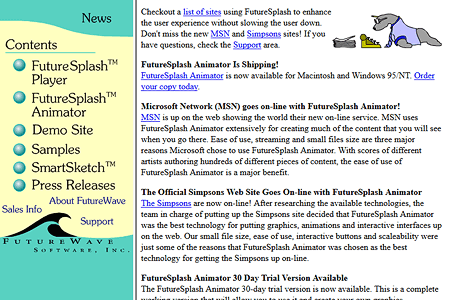The image displays the homepage of FutureWave Software Incorporated's website, characterized by a simplistic yet distinct design. The left side features a green motif, with a wavy green border at the top and a double wave, one large and one small, at the bottom, all in green. The company's name, "FutureWave Software Incorporated," is prominently displayed with "FutureWave" at the top and "Software Incorporated" beneath it.

In the left column, titled "Contents," a green line and bullet-point bubbles outline various sections. The bullet points list "Future Splash Player," "Future Splash Animator Demo Site Samples," "Smart Sketch," "Press Releases," "Sales Info" for contact inquiries, "Support," and "About FutureWave" for more information.

The right column contains a block of text encouraging viewers to explore sites utilizing Future Splash. It mentions clickable links for further details and highlights notable examples such as MSN and The Simpsons websites. A quirky illustration of an animal in a suit and glasses is also present, though its exact species is unclear. The animal is depicted looking at a keyboard, adding a whimsical touch to the page.

Underneath, a banner reads, "Future Splash Animator Shipping," with options to download the Animator for Mac or Windows 95, indicating the software's vintage. Additional text highlights that the Microsoft Network (MSN) and the official Simpsons website have both gone online using Future Splash Animator, providing context and significance to the software. The page concludes by offering a 30-day free trial for skeptical users who may need convincing before purchasing.